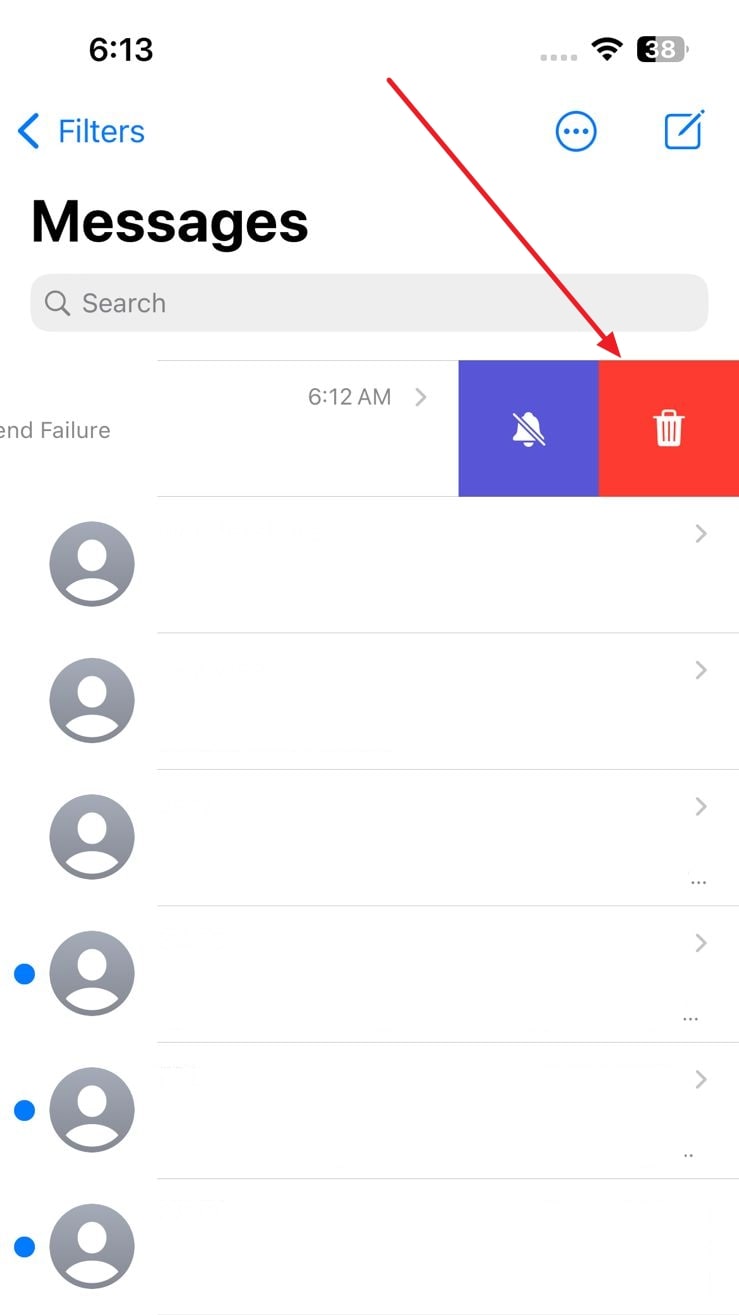The image displays a phone's messaging app interface, characterized by its white background and gray user icons. In the main view, there are no text messages visible. At the top of the screen, a search bar is present, though it currently shows no search results.

Below the search bar, six user icons are vertically aligned on the left side of the screen, all without associated names. The first three user icons are plain, while the last three each feature a blue dot on their left side, indicating unread messages. To the right of each icon is a right-pointing arrow suggesting navigation to a detail view.

Above the user icons, a truncated message displays "something failure," indicating a partial error message. More to the right, the time "6:12 AM" is shown. Adjacent to this, two boxes are aligned: one blue and one red. The red box has a muted icon and a trash can symbol with a red border. There is an arrow pointing diagonally down from the top right to the red box, indicating an action toward the trash can.

Above these elements, there is a blue "Filter" option and a left-pointing arrow for navigation. On the far right, three vertical dots within a circle and a square with a pencil icon suggest additional settings and the option to start a new message.

At the very top of the screen, the status bar shows the battery at 38%, full Wi-Fi signal, and the time "6:13." Overall, the interface is predominantly white, with gray user icons and highlighted areas in blue and red.